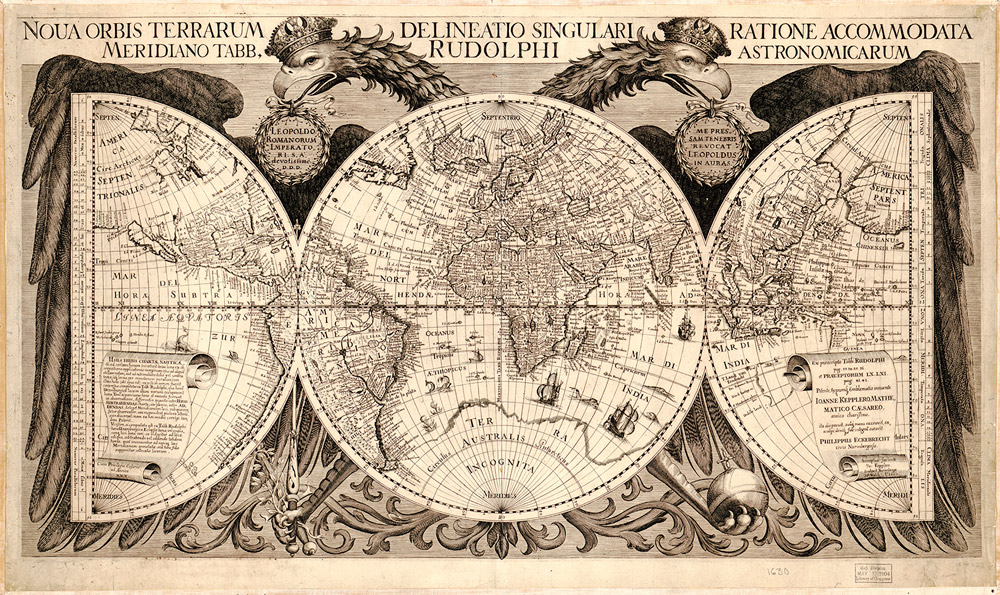This horizontally-oriented photograph depicts an antique world map that appears to be several centuries old, possibly a copy of an original from three to four hundred years ago. Central to the image is a large, round map representing the entire globe. Flanking this central globe are two hemispheres, each displaying additional continents. 

The map is adorned with numerous intricate lines and ornate decorations. At the top, there are Latin inscriptions which read: "Noah, Orbis, Terrarium, Nel Delanato, Singulari, Rationae, Accommodata." Positioned directly below the text, but above the globes, are images of two bird heads with elongated necks and beaks, each facing outward (one to the left and one to the right). Beneath these beaks are small, circular areas filled with text.

Below the globes, the map features ornate designs including filials, filigree, and feathers. The entire composition is framed by a thin white border, which has yellowed with age, complementing the overall antiquated appearance of the map.